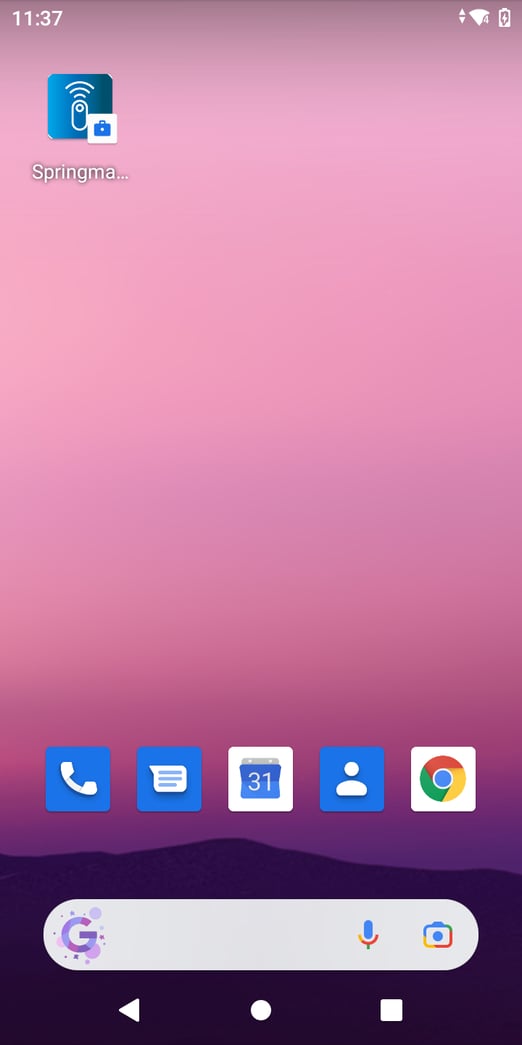This is a detailed screenshot of a smartphone screen taken at 11:37 AM. The top-left corner displays the time in white numbers, while the top-right corner features several icons including a wireless signal icon, a cellular service icon, and a white battery icon. Below these icons, "Spring MA" is displayed alongside a blue suitcase icon in a white box, whose significance is unclear.

The background of the screen transitions from pink at the top to purple at the bottom, creating a gradient effect reminiscent of a mountain silhouette at the base. Positioned above this shadowy mountain landscape are several app icons arranged horizontally. From left to right, they include:

1. A white phone icon inside a blue box.
2. A chat bubble icon inside a blue box.
3. A calendar icon displaying the number "31" inside a white box.
4. A profile icon of a person inside a blue box.
5. The Chrome browser icon inside a white box. 

Below this row of icons, a purple Google "G" with surrounding bubbles is prominently displayed. Adjacent to this, and further right, a blue microphone icon and a camera icon are visible, separated by some empty space.

At the very bottom of the screen, the navigation bar features three white icons: a left-pointing arrow on the left, a circular home button in the center, and a square button on the right.